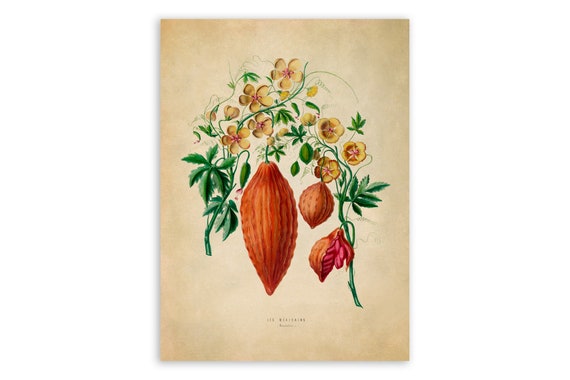This image showcases a detailed drawing on a rectangular canvas with an antique, beige-yellow background. Dominating the scene is a green vegetable vine that spans from the left side, arches over the top, and descends to the right. Hanging prominently from the vine are three long, cylindrical vegetables of a dark reddish-orange color. The vine is adorned with flowers featuring 2 to 5 petals, varying in number, and displaying shades of gold to beige-yellow. Green leaves sprout abundantly along the vine, enhancing the natural feel of the composition. At the bottom center of the canvas, there is some small, illegible black text.